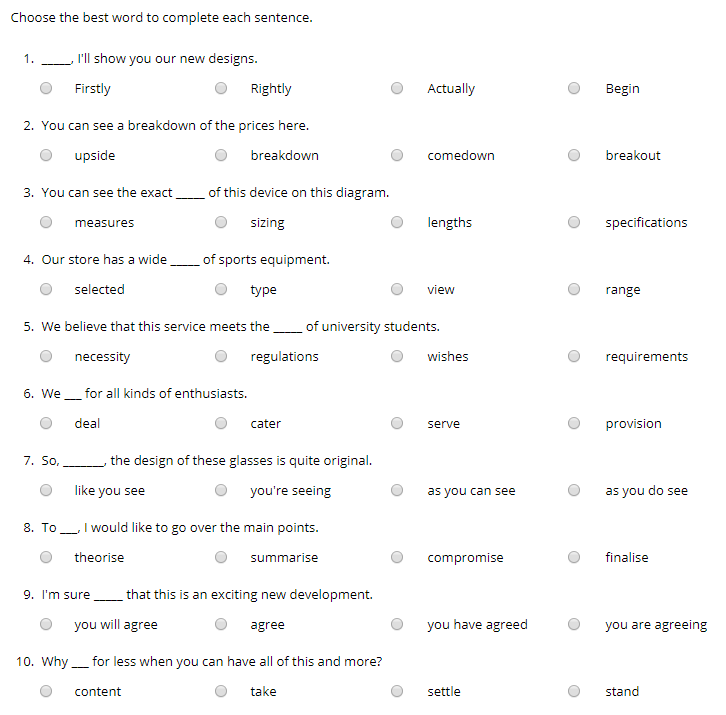The image features a white background with a series of sentences where you choose the best word to complete each. The task appears in a single line with the instruction, "I'll show you our new designs," followed by a series of four options for each sentence. The options are presented in four circles, each corresponding to a different blank in the sentences. 

1. Firstly, rightly, actually, begin.
2. Can you see a breakdown of the prices here? Upside, breakdown, come down, breakout.
3. You can see the exact measures, sizing, lengths, specifications of this device on this diagram.
4. Our store has a broad range of sports equipment. Selected, type, view, range.
5. We believe that this service meets the requirements of university students. Necessity, regulations, wishes, requirements.
6. We cater for all kinds of enthusiast. Deal, cater, serve, provision.
7. So, the design of these glasses is quite original. Like you see. 

Each sentence has a blank to fill, and the completion options are provided in circles. This setup helps to guide the user in selecting the appropriate choice to complete each sentence correctly. The aim is to showcase the new designs and explain their features through a clear and interactive visual.